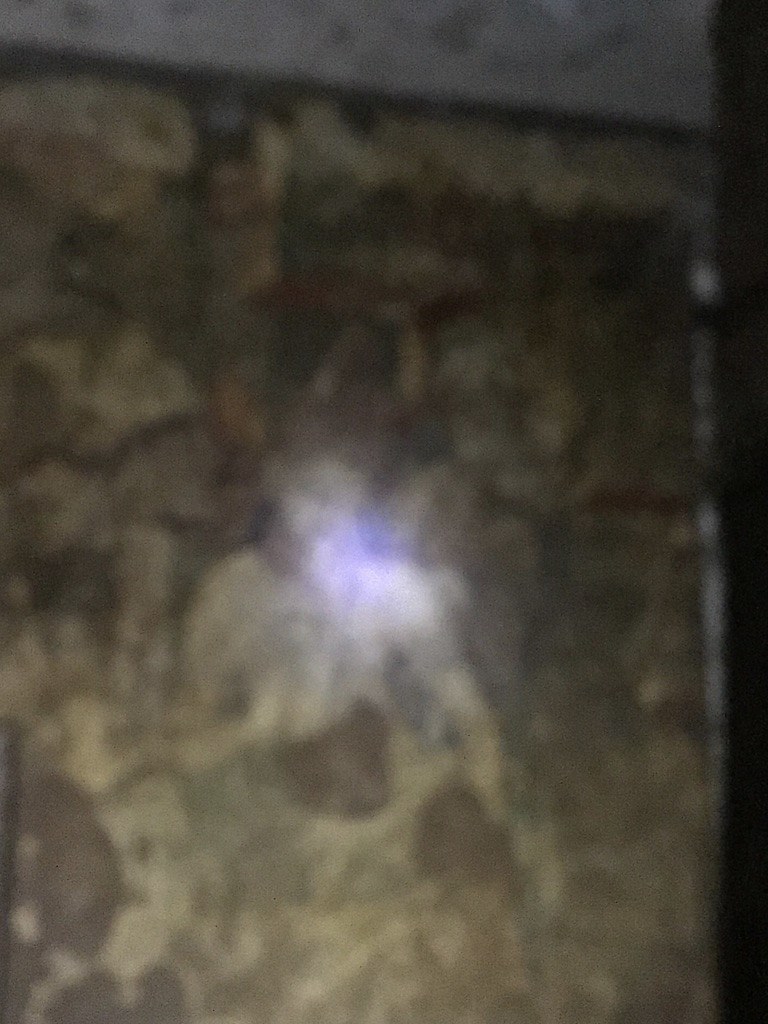The image showcases a blurry and complex surface, possibly a wall, poster, or painting, with an unclear subject. It features a predominantly dark and mottled color palette, including shades of brown, tan, gray, and brick red. There is a prominent horizontal dark line across the top. Near the center, light reflects off a shiny, polished surface—potentially glass—resulting in bright whites, blues, and purples. Some viewers suggest the image might depict a human figure with floral or leafy patterns around it, possibly a tapestry under glass. The right side has a notable dark vertical bar, and there are several round brown spots toward the bottom. Above the dark line, the image lightens to an off-white or lighter gray color.